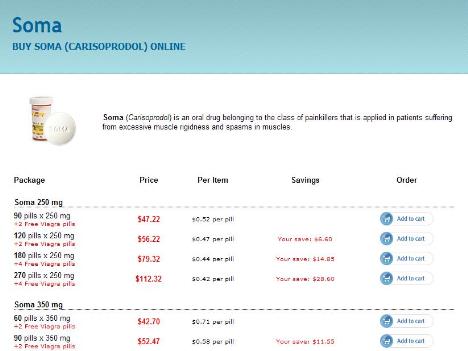The image is a vertically-oriented screenshot of a pharmaceutical website, likely viewable on a smart device or a computer. The background predominantly features a clean white space, leveraging the screen's natural color. At the top, a seafoam green navbar stretches horizontally, displaying various shades of the color to add a sense of dimension. On the left-hand side of this navbar, the word "Soma" is prominently displayed in bold blue font.

Beneath the logo, smaller text reads "Buy Soma, Karius, So Protal, Online." Below this header, the image transitions to a white background displaying a pill bottle alongside a close-up, enlarged view of a single pill. The bottle label, SIOMA, is clearly visible.

Further down, descriptive text appears. It identifies Soma as an oral medication belonging to a class of painkillers designed to relieve patients experiencing severe muscle soreness and spasms. Additional details outline the package dosage, price per item, potential savings, and purchasing options. On the right-hand side, there is an "Add to Cart" button, facilitating easy online purchase of the drug.